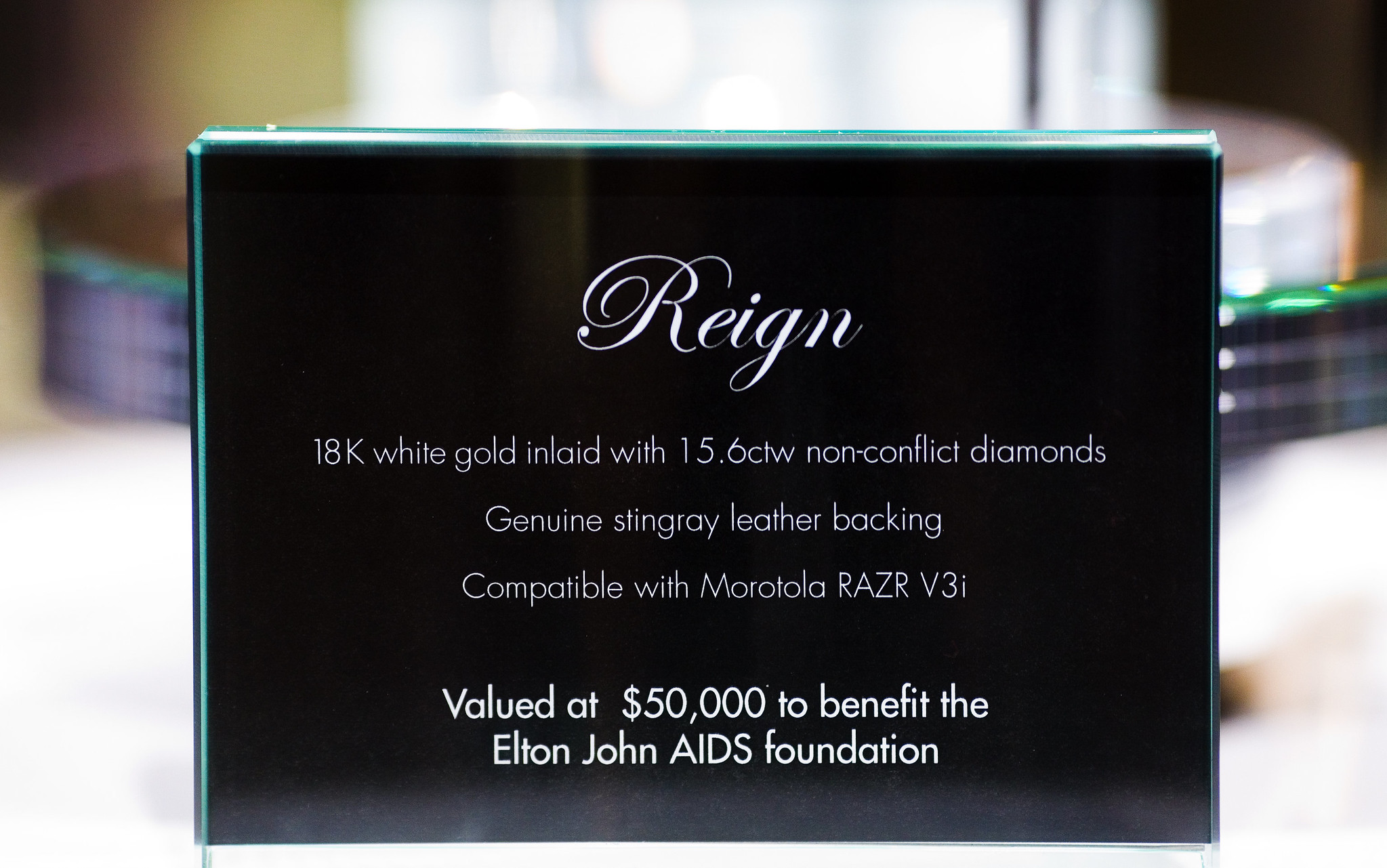This colorful photograph captures a close-up of a small, square informational plaque nestled within a sleek, clear acrylic case designed for displaying paper items. The focal point is a tiny rectangular black card with pristine white text that reads: "Rain, 18 karat white gold inlaid with 15.6 CTW non-conflict diamonds. Genuine Stingray leather backing, compatible with Motorola RAZR V3i. Valued at $50,000 to benefit the Elton John AIDS Foundation." Behind the plaque, on a slightly blurry pedestal, there appears to be a white cylindrical object, possibly housed in a white case, lending an air of mystery to the sophisticated display. Overall, this image showcases a luxurious and charitable offering prominently set in a jeweler's display case.